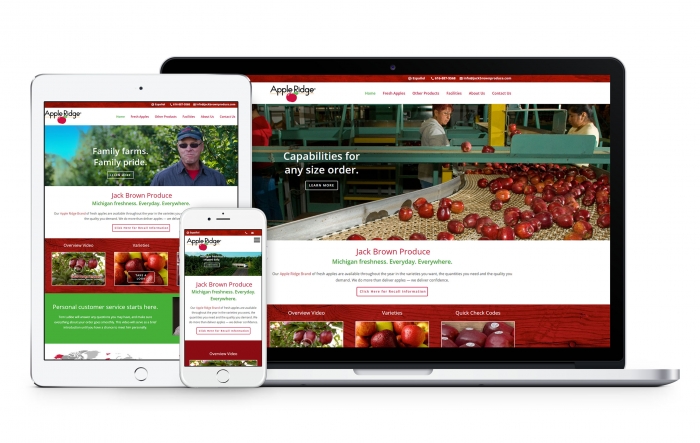In this photo, we see a detailed digital representation showcasing the Apple Ridge website across multiple devices: a laptop, an iPad, and a phone. Each device is prominently displayed against a minimalist white background, highlighting the core content without distractions.

The backdrop of the webpage features a blend of white and red hues, creating a visually appealing contrast. At the top of the webpage, a red banner is noticeable on all screens, providing a cohesive design element across the devices.

On the laptop screen, the website displays an engaging image of apples being neatly organized on an assembly line within a factory setting, emphasizing the precision and care in the production process. 

The iPad screen captures a more agricultural scene, with a man standing outdoors, framed by large, lush bushes. This image conveys the hands-on approach and natural environment of Apple Ridge.

Meanwhile, the phone screen offers an overhead view of the expansive Apple Ridge area, showcasing the vastness and scale of the farm.

Each device prominently features the text "Jack Brown Produce" in bold red letters on a white ribbon that runs across the middle of the webpage. Below this, the tagline "Michigan, some freshness every day, everywhere" is displayed, reinforcing the commitment to quality and freshness that the brand stands for.

The arrangement and the consistency across devices highlight the versatility and user-friendly interface of the Apple Ridge website, making it accessible and appealing on any platform.